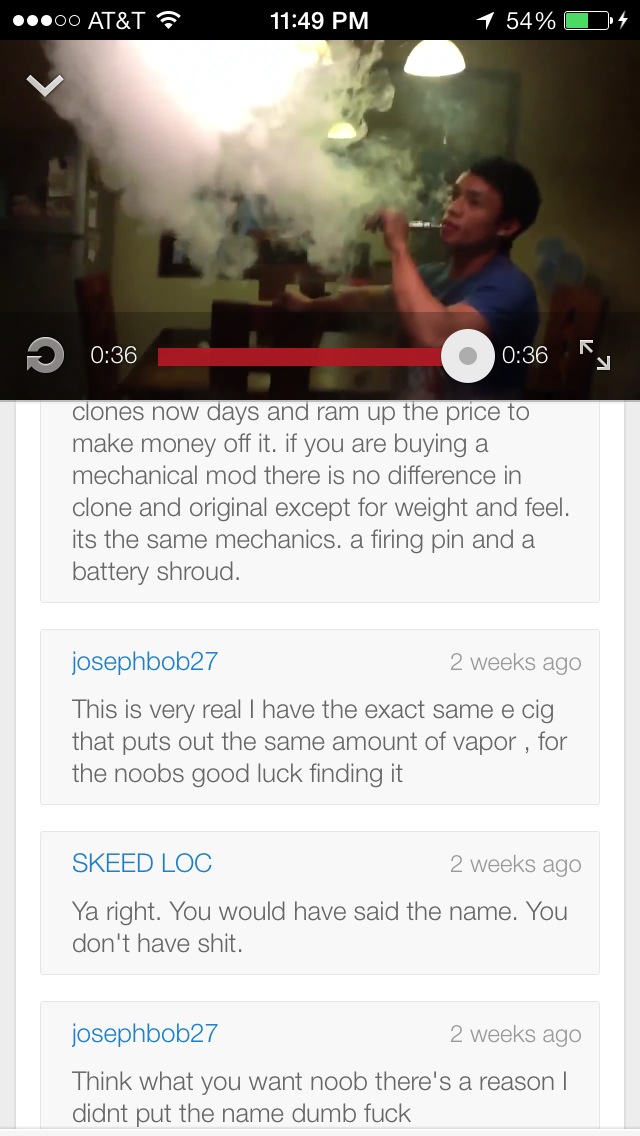This is a detailed screenshot of a smartphone screen showing a paused video of an individual vaping from a pen, shrouding their face in a dense cloud of smoke. The video is framed at the top with a status bar indicating it's 11:49 PM, the service provider is AT&T, the Wi-Fi is connected, and the battery is at 54%, depicted by a green battery icon. The person's name is Joseph Bob, age 27, with the username "Skidloak." Surrounding this small 36-second video, which features an Asian man, possibly with a mirror or a large picture in the background, are several user comments. The primary comment thread below the video discusses the cost differences between original and clone mechanical mods for vaping, making a point that there is no functional difference apart from weight and feel. Additional comments from three different users, dated two weeks ago, further engage with this topic. The video player is accentuated by a red progress bar at the bottom, indicating the video has reached its end.